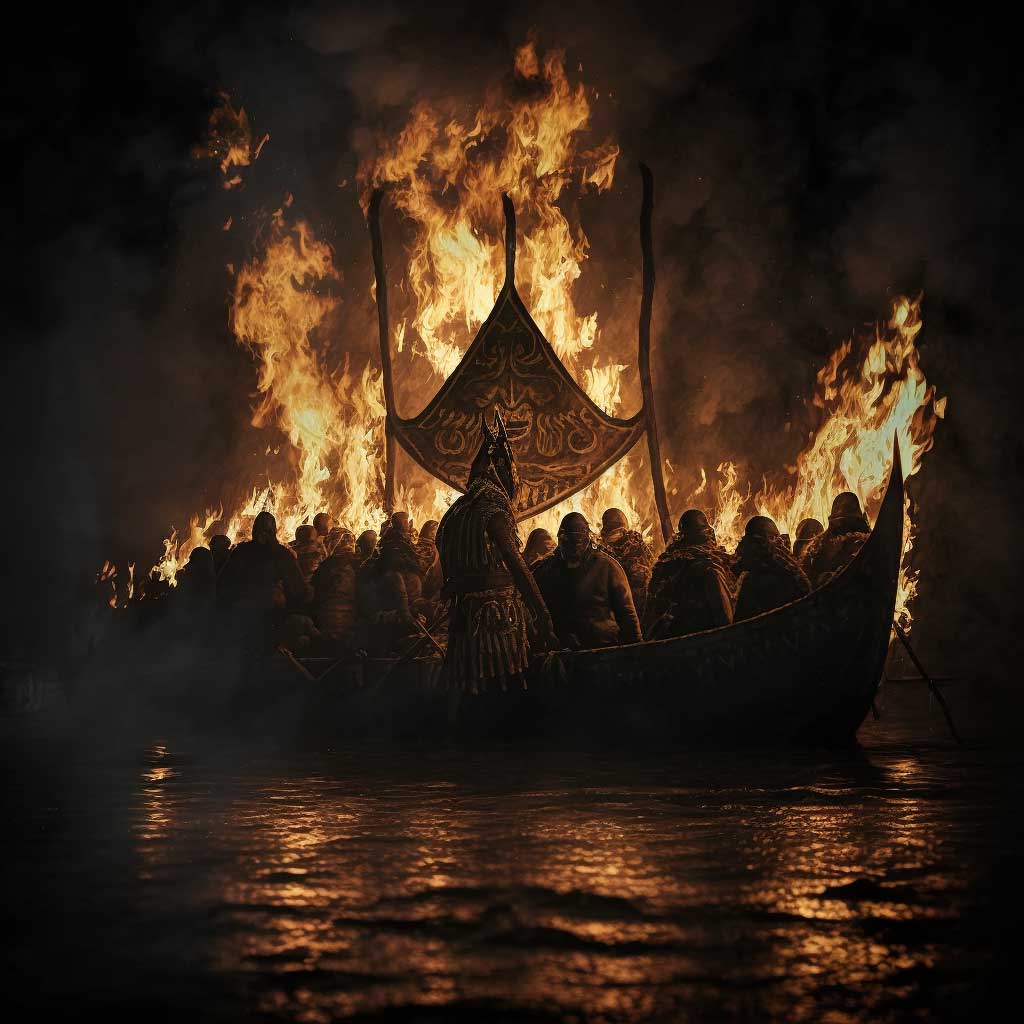A captivating, highly detailed painting depicts a dramatic night scene featuring Viking warriors seated in an old-school canoe navigating through shallow waters. Positioned prominently in the foreground, the boat is adorned with a large, abstract banner or logo, supported by three wooden columns. The calm water mirrors the fierce blaze dominating the background. The fire, with its intense reds, oranges, yellows, and dark browns, engulfs another structure, likely another boat, creating a stark contrast against the night sky. The warriors, all facing the massive, towering flames, add depth and emotion to the scene, capturing a moment of intense focus and reflection. The artwork's realism is striking, particularly in the reflections of the fire on the serene water's surface.